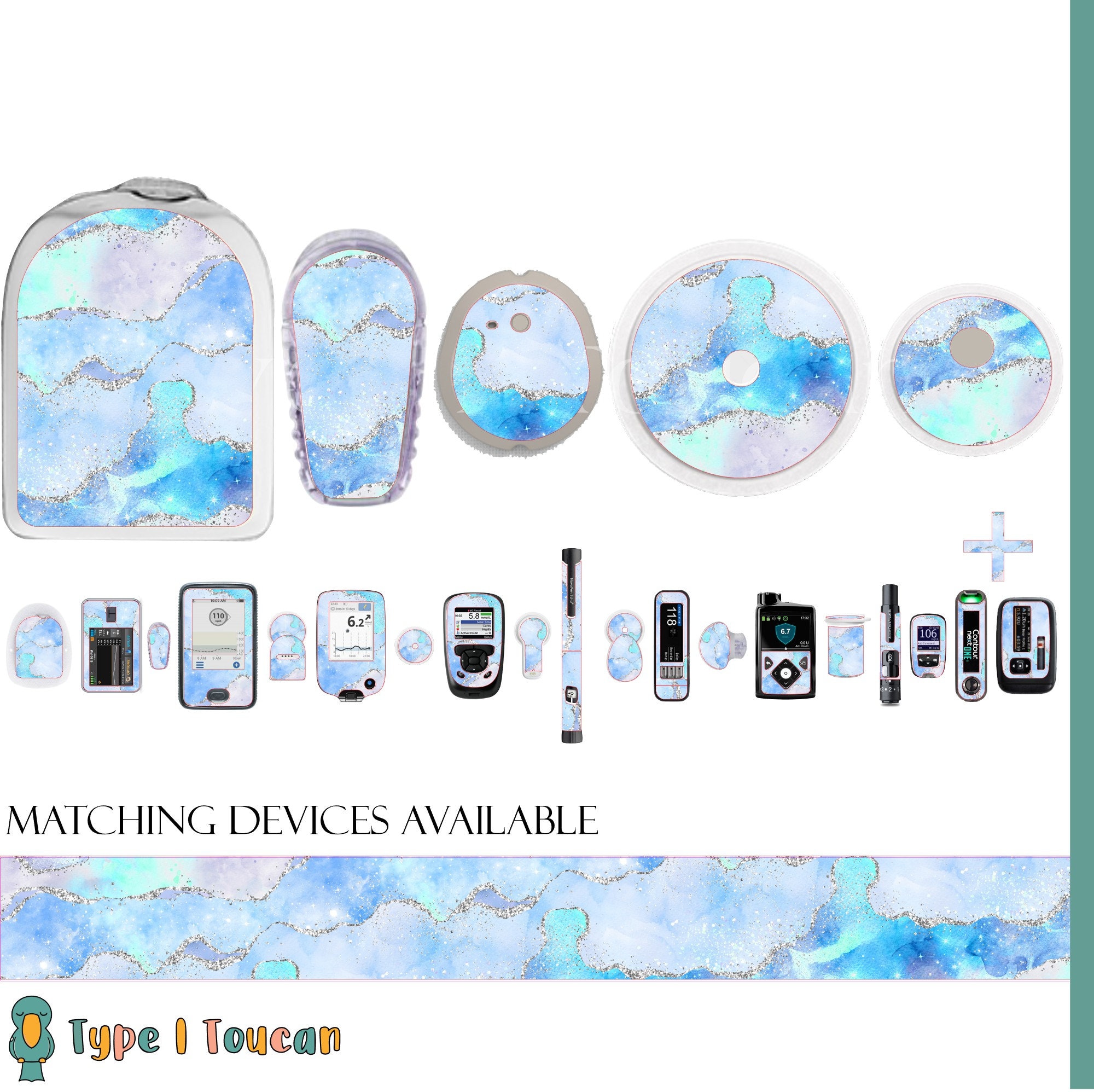The image depicts a professional promotional advertisement for Type 1 Toucan, featuring a variety of handheld medical devices, primarily glucose and oxygen meters, all adorned with a distinctive blue marble pattern. The top section displays a collection of shapes with the same marble design, including round, oval, and disc-like forms, suggesting customizable skins that can be applied to different gadgets. Specifically, the shapes showcased range from something resembling a mailbox's interior to ones akin to the bottom of a mouse, a CD with a central hole, and spherical objects with gray dots. The middle section illustrates various medical devices with this marbled design overlay, indicating their practical usage. Among these are blood sugar measurement tools, an odometer, small and large phones, a measuring device, a pen-like object, and different sizes of MP3 players. The bottom section highlights a rectangular banner in blue marble pattern with the text "Matching devices available" accompanied by the brand name, Type 1 Toucan. The overall presentation is vibrant and engaging, emphasizing the cohesive design across numerous devices.